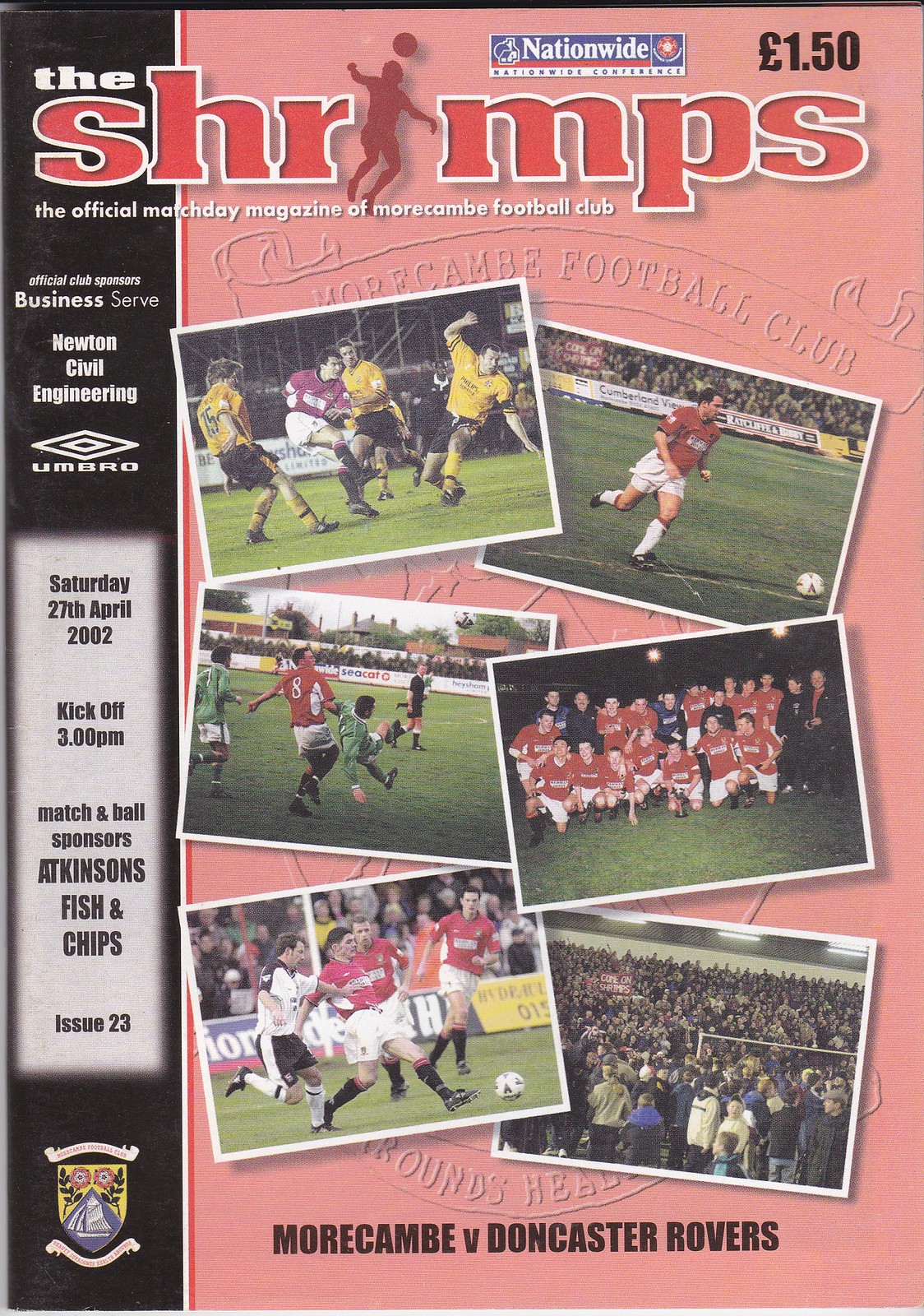The cover of the magazine is an advertisement for the official match day magazine of Morecambe Football Club. Dominating the top section, the title "The Shrimps" is prominently displayed in bold red letters with a white outline, with the letter 'I' cleverly designed as a silhouette of a man bouncing a ball off the top of his head. The upper right corner has the price listed as £1.50, accompanied by a rectangle logo for Nationwide. Below the title, in white text on a light pink background, it reads "The Official Matchday Magazine of Morecambe Football Club."

The cover's right side features a pastel red graphical motif, while a black bar runs down the left side containing several white text elements. It lists the official club sponsors: Business Serve, Newton Civil Engineering, and Umbro, followed by details of the match day: "Saturday, 27 April 2002, Kickoff, 3 p.m. Match and ball sponsors: Atkinson's Fish and Chips, Issue 23."

The main section showcases six photographs of various match scenes:
1. The upper left image displays four soccer players—three in yellow jerseys and one in a red jersey.
2. To the right, another photo highlights a single player in a red jersey on a soccer field, ready to kick a soccer ball.
3. In the middle left, a striking action shot shows a player in a red jersey (number 8) amidst green-jerseyed opponents.
4. Adjacent to it, the entire soccer team is seen posing in two rows with players mostly in red jerseys, some in black coats or blue jerseys.
5. The bottom left image captures three men in red jerseys and one in a white jersey all vying for the ball.
6. Lastly, the bottom right photo provides an overhead view of a crowded stadium.

At the very bottom in black text, the cover mentions the matchup: "Morecambe vs. Doncaster Rovers." The black bar on the left further reiterates the event details and sponsors, ensuring a comprehensive presentation.